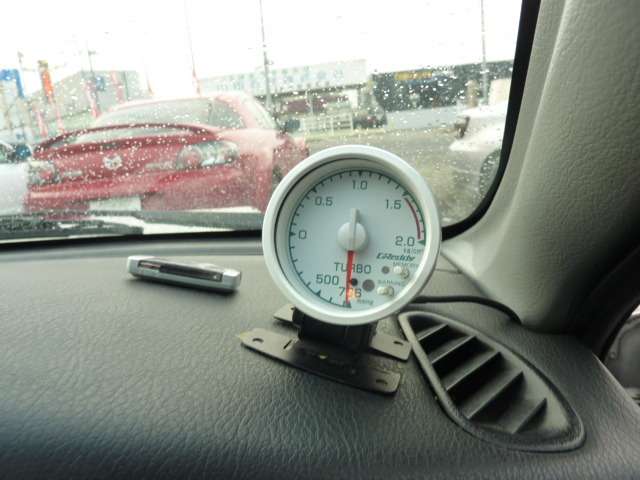A detailed color photograph captures the interior of a vehicle, focusing closely on the right side of the dashboard in front of the passenger seat. The main feature of this scene is a round gauge with a glass cover, prominently displayed on the dashboard. The gauge has a white face and features a red needle attached to a central white hub. The dial is marked with the word "Turbo" positioned directly beneath the central hub. Numerous numerals are displayed around the edge of the dial, which also has a green line with hash marks. The numbers range from 2.0 at the upper right (around the 2 o'clock position), to 1.0 at the top center (12 o'clock), 0 on the left side (9 o'clock), then escalating sharply to 500 and reaching 796 at the bottom (approximately 6 o'clock), where the red needle currently points. The gauge itself is set in a steel base that appears to allow screwing in but is not presently secured to the dashboard. Through the windshield, raindrops are visible, with a red sporty car faintly seen ahead, completing the vivid and dynamic scene inside the vehicle.